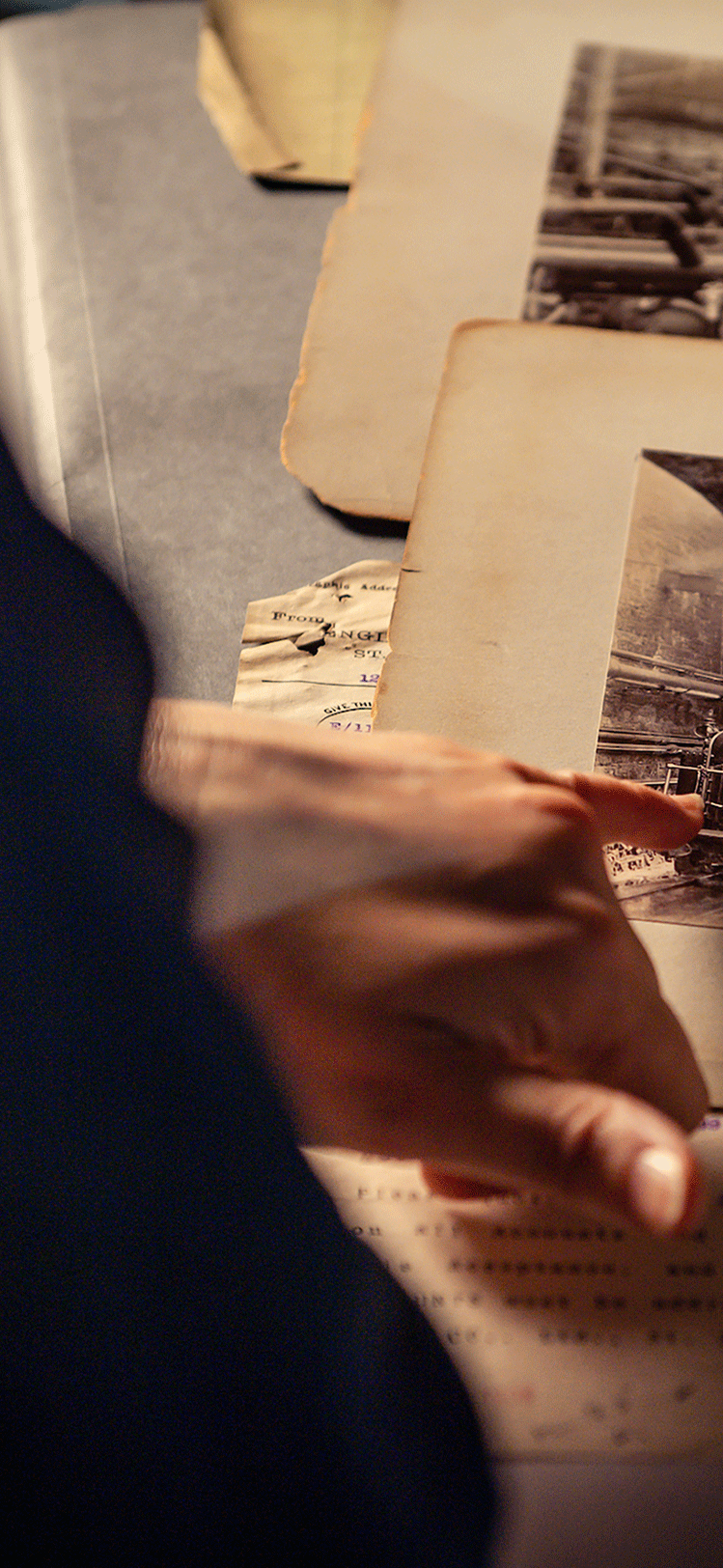The image captures a close-up of a light-skinned Caucasian hand, likely male, pointing delicately with the pinky and thumb extended, at an old, weathered photograph. The hand appears to belong to someone standing slightly to the back, with part of a dark-clad shoulder or arm visible in the bottom left, casting a shadow. The photograph being pointed to is indistinct but clearly aged, perhaps from the early 1900s, displaying signs of wear such as crinkles and tears. Behind this photo lies another similarly aged photograph. Beneath these images rests a document or manifest, featuring blue stamps and dates, suggesting historical significance. The overall scene conveys a sense of nostalgia and historical intrigue.